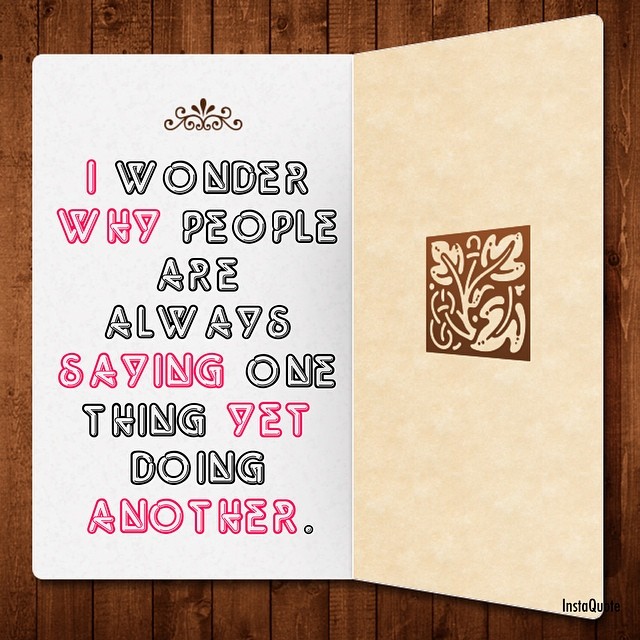The image showcases an open paper card resting on a dark brown wooden surface with visible wood panels in the background. The left page of the card is white, while the right page is a tan, off-white, or yellowish color. In the center of the right page, there is a small square design featuring a pattern of twisting vines and leaves in brown. On the top of the left page, there is a small ornamental symbol, followed by a phrase in white text bordered either by pink or black. The text reads, "I wonder why people are always saying one thing yet doing another." The sentence concludes with a black period.